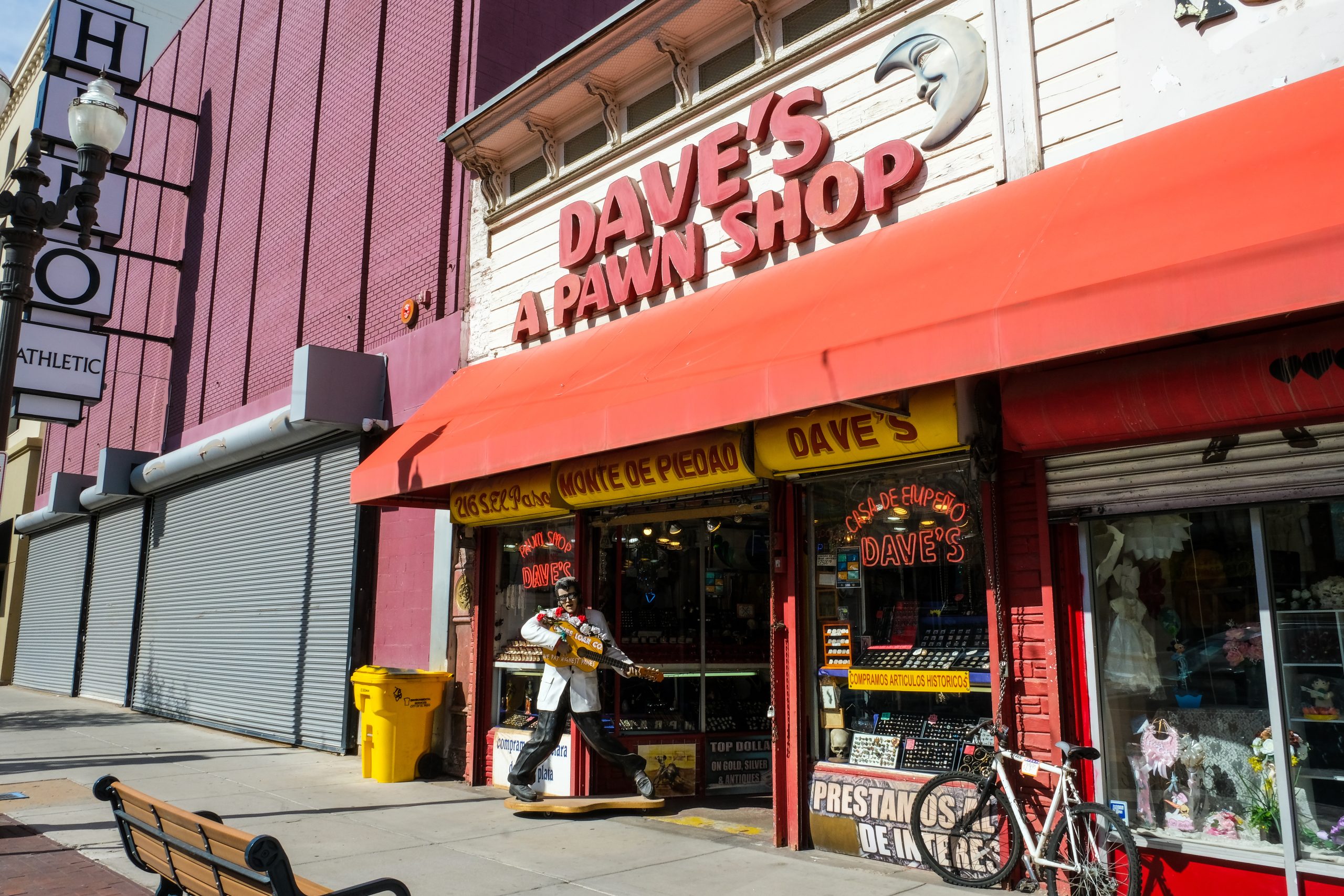The image captures a bustling city sidewalk scene, showcasing the exterior of Dave's Pawn Shop. Dominating the top center of the photo, the store's signboard features bold, red capital letters reading "Dave's" above "Pawn Shop," with a smiling crescent moon symbol to the right. The storefront itself is adorned with an orange canopy and a white upper level, which boasts horizontal siding.

In front of the shop stands an Elvis Presley statue, striking a classic pose with bent knees and separated legs, dressed in a white jacket and holding a guitar. To the left of the pawn shop is an adjoining building with grey metal shutters and a vibrant pink facade, separated by a yellow garbage can. Leaning against the store is a white bicycle with black tires.

The window of Dave's Pawn Shop features a neon sign and Spanish text, which partially reads "Casa de Impero Dave's". Items like jewelry are displayed on shelves facing the viewer through the glass. Adjacent to this, a red storefront displays children's clothing. Further details include a brown and black bench, a streetlamp, and various colorful signs, including one vertical sign for "Hero Athletic" partially obscured by a streetlight.

The scene is rich with color and texture, including hues of gray, tan, brown, black, white, red, yellow, purple, green, and orange, encapsulating a vivid representation of urban life and commercial activity.